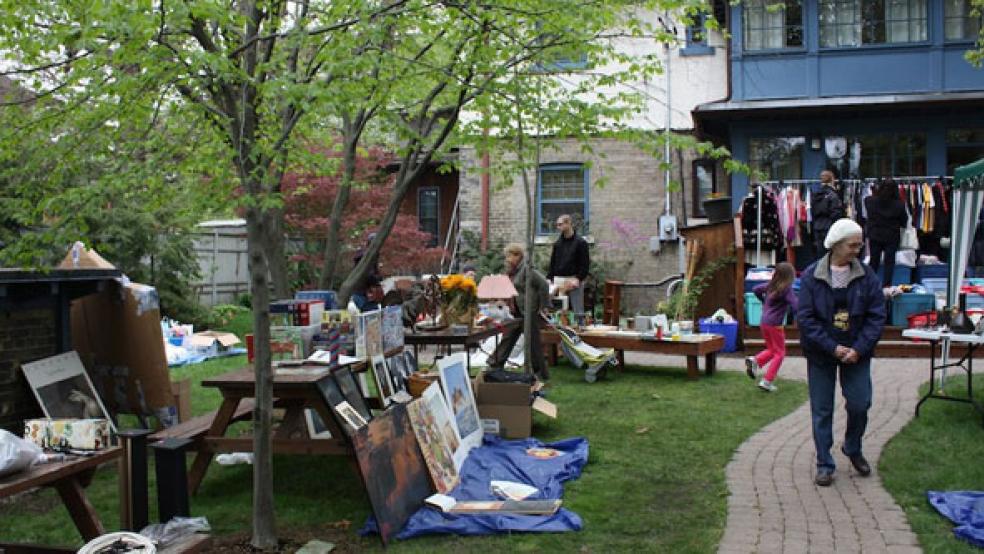This photograph captures an outdoor yard sale set in the courtyard of an apartment building. In the background, several buildings with brick, white, and blue facades create a colorful backdrop. A blue building stands out, where clothing racks are prominently displayed. The courtyard is adorned with a blue tarp, on which numerous paintings and framed photographs are carefully arranged for display. These artworks lean against a variety of surfaces, including picnic tables and benches, possibly even on the grass. The yard sale also features various household knickknacks, lamps, and books, creating a vibrant, eclectic scene. Several people are milling about, inspecting the items; a couple focuses on the clothes, while another pair examines the art. Among the shoppers is an older woman in a white hairnet or beret walking along a pathway that cuts through the green space. The scene is further enriched with trees—the vibrant reds of autumn leaves in the background adding color contrast, while lush green leaves in the foreground complete the picturesque setting. It appears to be either a summer or fall day, likely in a northeastern locale, based on the foliage and overall atmosphere.